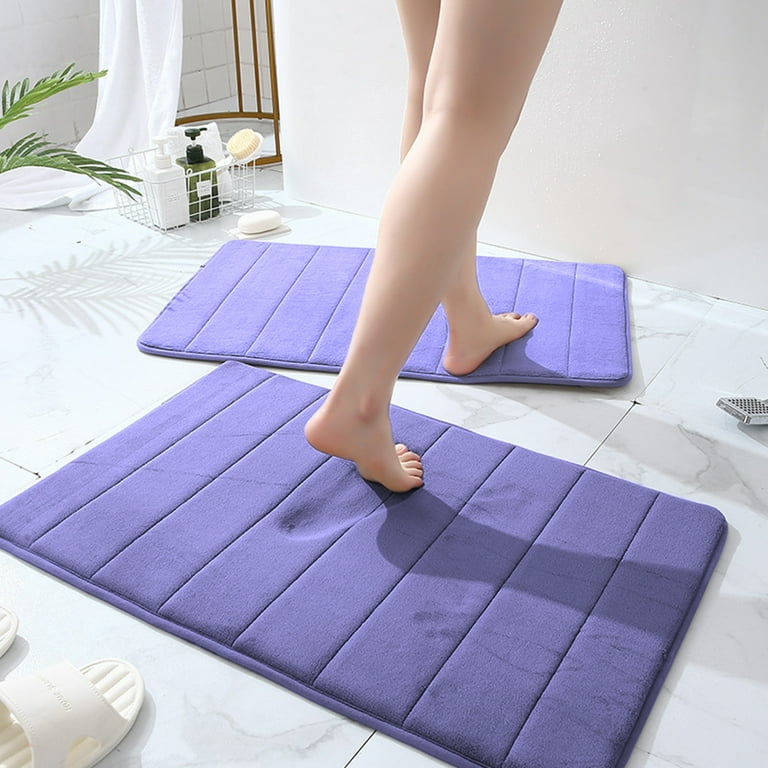The image depicts a woman standing in a bathroom area on two large, purple microfiber and memory foam bath mats placed on a white tiled floor with a subtle gray wavy pattern. Her legs are visible from the mid-thigh down, with her left foot planted flat on the front mat and her right foot slightly lifted on the back mat, leaving a prominent footprint on the rear mat, indicating the plush, memory foam texture. To the bottom left of the image, a white sandal, typically used for a sauna or bath, is casually placed on the floor. In the top left corner, part of a lush green plant is visible alongside a white shower caddy that contains various items, including a green pump-top bottle and a white pump-top bottle. Additionally, there are indications of a soap bar placed within or near the caddy, reinforcing the bathroom setting. The overall scene suggests a calm and tidy restroom environment, emphasizing both the comfort and functionality of the space.